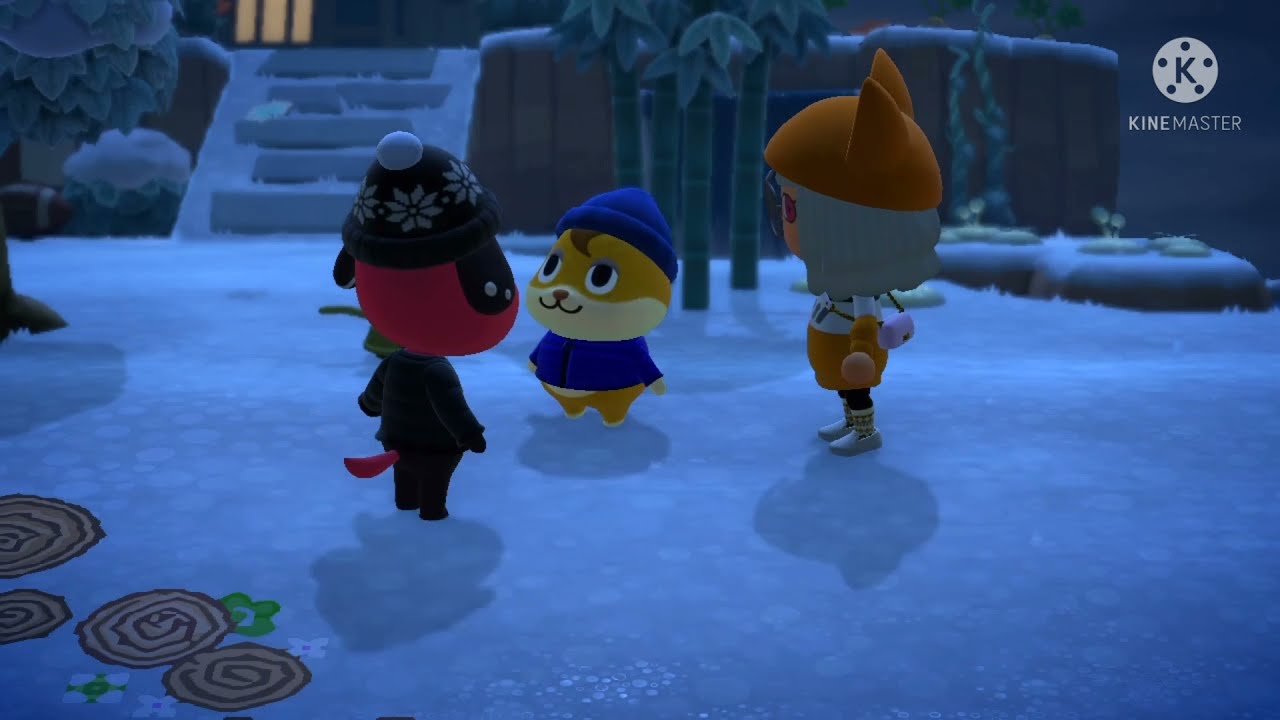In the image, a scene from what resembles the animation style of Animal Crossing is depicted, where three characters are interacting in a snowy environment. In the center, a dog-like figure wearing a knit winter hat adorned with snowflakes and a blue jacket stands. Beside it is another dog-like creature, distinguishable by its blue knit cap and matching jacket. The third character is a human-like figure with white hair and skin, donning a hat with cat ears and a brownish sweater. They are all clustered together, seemingly engaged in conversation. The backdrop features bamboo stalks and a set of stairs ascending in the upper left corner. The scene is set at nighttime, adding a darker hue to the surroundings. Adding to the image's digital nature, the upper right corner bears the "KineMaster" logo, indicating it was captured or processed using that video editing software.